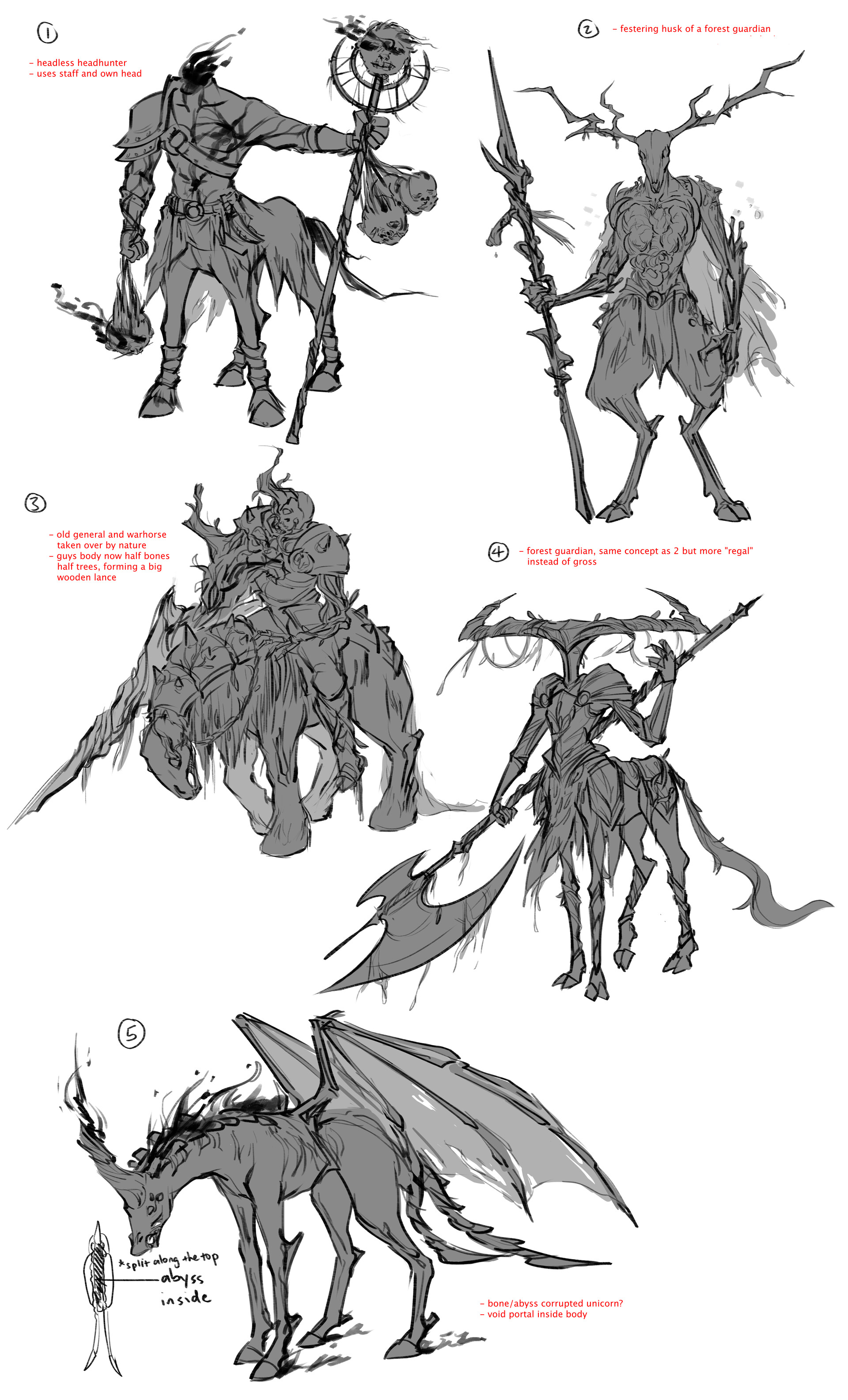A detailed concept art illustration features five numbered mythical characters set against a white background, primarily rendered in detailed black-and-gray sketches. Number 1, located in the upper left corner, is the "Headless Hunter," a creature with the body of a horse and a human upper body, dressed in colonial-like gear. It holds a staff with its own severed head attached in its left hand. Number 2, known as the "Festering Husk of a Forest Guardian," depicts a standing deer-like figure with a deer skull head and a demonic body, wielding a staff in its right hand. Number 3, labeled "Old General and War Horse," portrays a monstrous skeleton-like figure in armor, riding a diseased horse. This character holds a large weapon resembling a tree trunk spear. Number 4, another "Forest Guardian," shares similarities with number 2 but appears more regal, featuring a longer head, extended antlers, and a massive battle axe. Number 5, labeled "Bone Abyss Corrupted Unicorn," is a skeletal unicorn with dragon wings and dual tails, embodying a dark, corrupted essence.